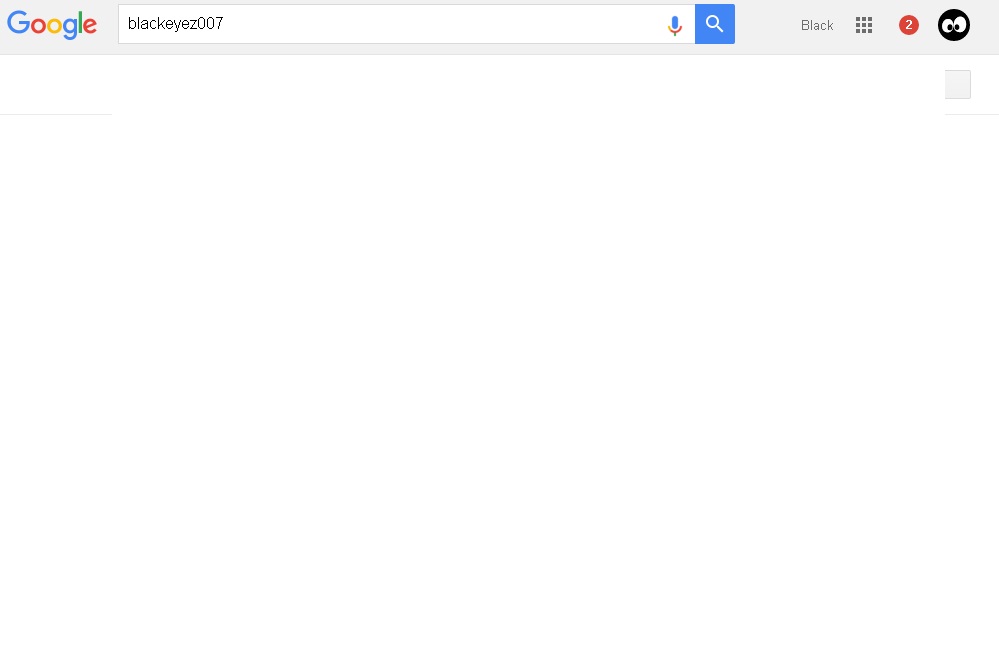The image depicts a Google search page. In the upper left corner, the Google logo is prominently displayed, with each letter in the logo colored distinctly: the capital 'G' in blue, the first lowercase 'o' in red, the second 'o' in yellow, the 'g' in blue, the 'l' in green, and the 'e' in red. Immediately to the right of the logo, there is a prominent white search bar where the term "BLACKEYEZ007" has been typed. To the right of the search bar, there is a microphone icon followed by a blue square search button with a magnifying glass icon inside it.

Further to the right of the search bar, the word "black" appears, next to a grid icon comprising three rows and three columns of dots. Continuing rightward, there is a red circle with the number '2' inside, indicating some form of notification. Beside it, a black circle features a minimalist face with two white eyes, each with small black pupils, suggesting a user profile or account menu.

Below this header region, the rest of the screen is mostly white, with a small gray square positioned in the upper right corner of the white space. The rest of the screen remains largely blank, emphasizing the central focus on the search bar and the header icons.